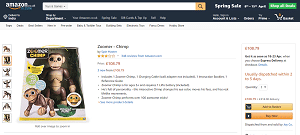The image depicts a section of an Amazon webpage, likely from the Spring Sale event, showcasing a toy monkey. The toy monkey features jointed limbs, allowing it to be posed in various positions. In the primary image, the monkey is seated on its rump, while a smaller thumbnail adjacent to it shows the toy in a crouched position, further emphasizing its poseability. Down the left-hand side of the webpage, there are additional images or possibly different versions of the toy, though the details remain unclear due to the extreme blurriness and small size of the image. Despite the lack of clarity, it is apparent that this page is dedicated to the sale of this poseable toy monkey.